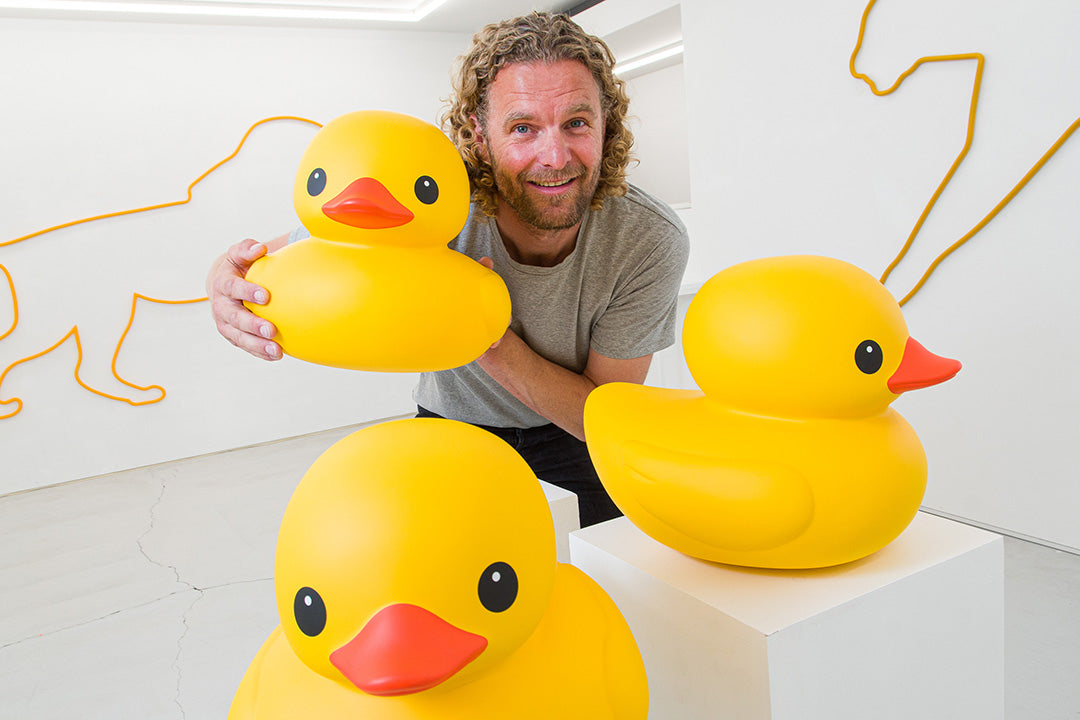In the image, a man with shoulder-length, sun-damaged light brown hair, which appears wavy and slightly curly, is posing in a gallery setting. He has a thin, trimmed beard and is dressed in a short-sleeve gray t-shirt and either black pants or dark blue jeans. He is holding a large yellow rubber duck with both hands, while two similarly large rubber ducks, about the size of a beach ball or twice the size of his head, are displayed on white wooden pedestals in front of him. The rubber ducks feature typical characteristics: bright yellow bodies, black eyes with small white reflective dots, orange beaks, and wings on either side. The gallery's walls and floor are white, adorned with yellow outlines of animals, including a tiger and a lion, adding an artistic flair to the setting. The man is smiling and looking straight ahead, creating a playful and cheerful atmosphere in the photo.